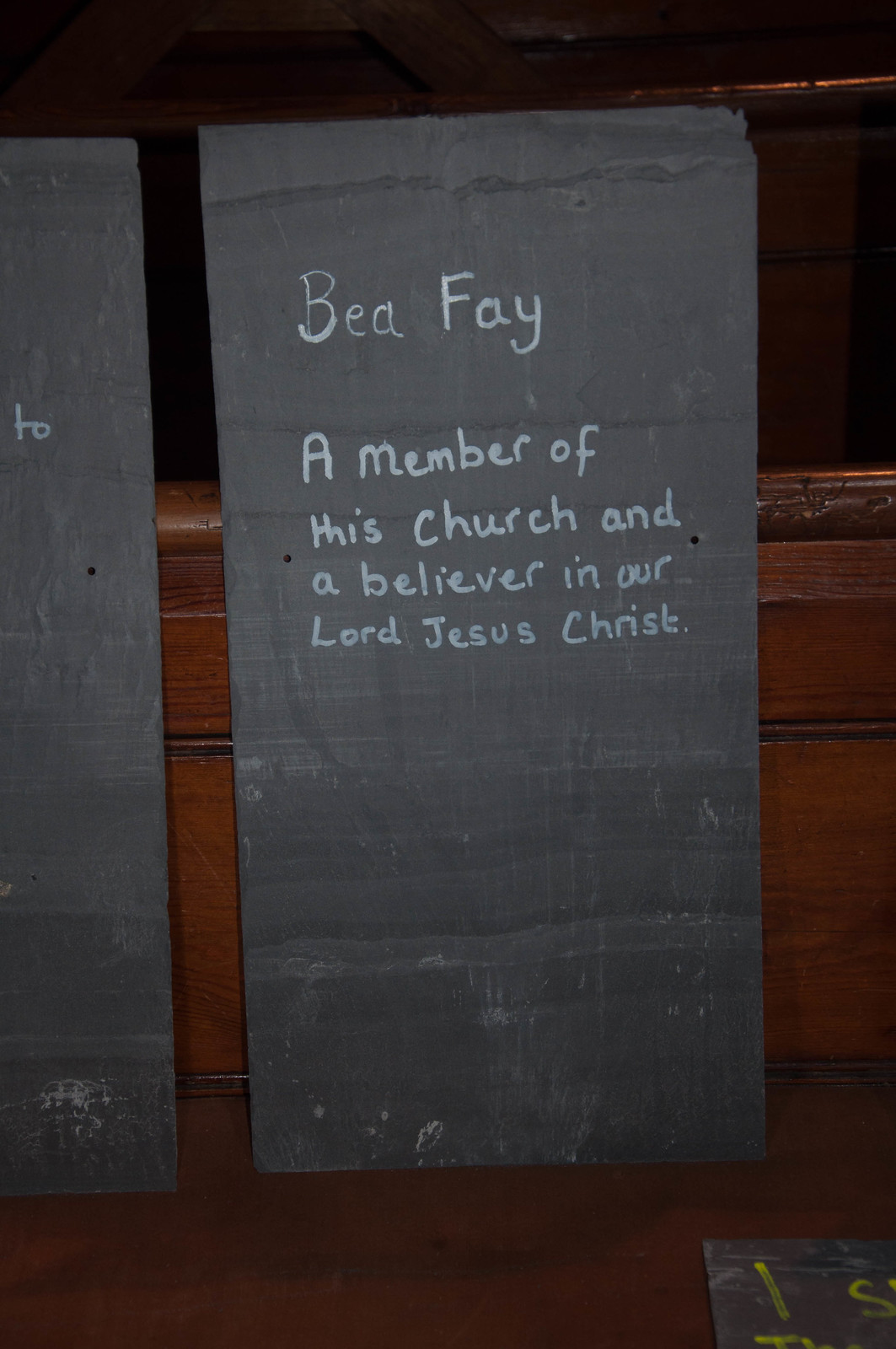The photograph features a large, vertically-oriented rectangular slate with a dirty gray appearance, hanging on an oak wall. The slate has white text, which reads, "B. Faye, a member of this church and a believer in our Lord Jesus Christ." The text is painted or written in white, occupying the top half of the slate, while the bottom half remains blank. Adjacent to it on the left, there is another similar slate with writing on it, although most of its text is illegible except for the word "to." The slates are positioned in what appears to be a church setting, possibly resting against a wooden pew or a bench.